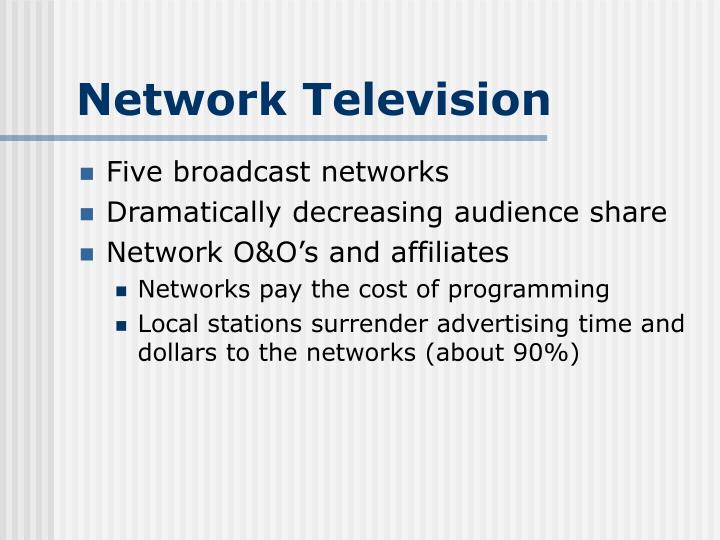The image depicts a well-organized presentation slide with a background consisting of vertical stripes in varying shades of gray. The title "Network Television" is prominently displayed at the top in dark navy blue text, underlined by a horizontal divider that separates the header from the main content. The slide is primarily text-based, featuring five bullet points in black. These bullet points outline the key points: "five broadcast networks," "dramatically decreasing audience share," "network O&Os and affiliates," "networks pay the cost of programming," and "local stations surrender advertising time and dollars to the networks (about 90%)." The layout is well-centered, and the color scheme includes shades of gray, blue, white, and black, enhancing readability. The slide is characteristic of a professional PowerPoint presentation.